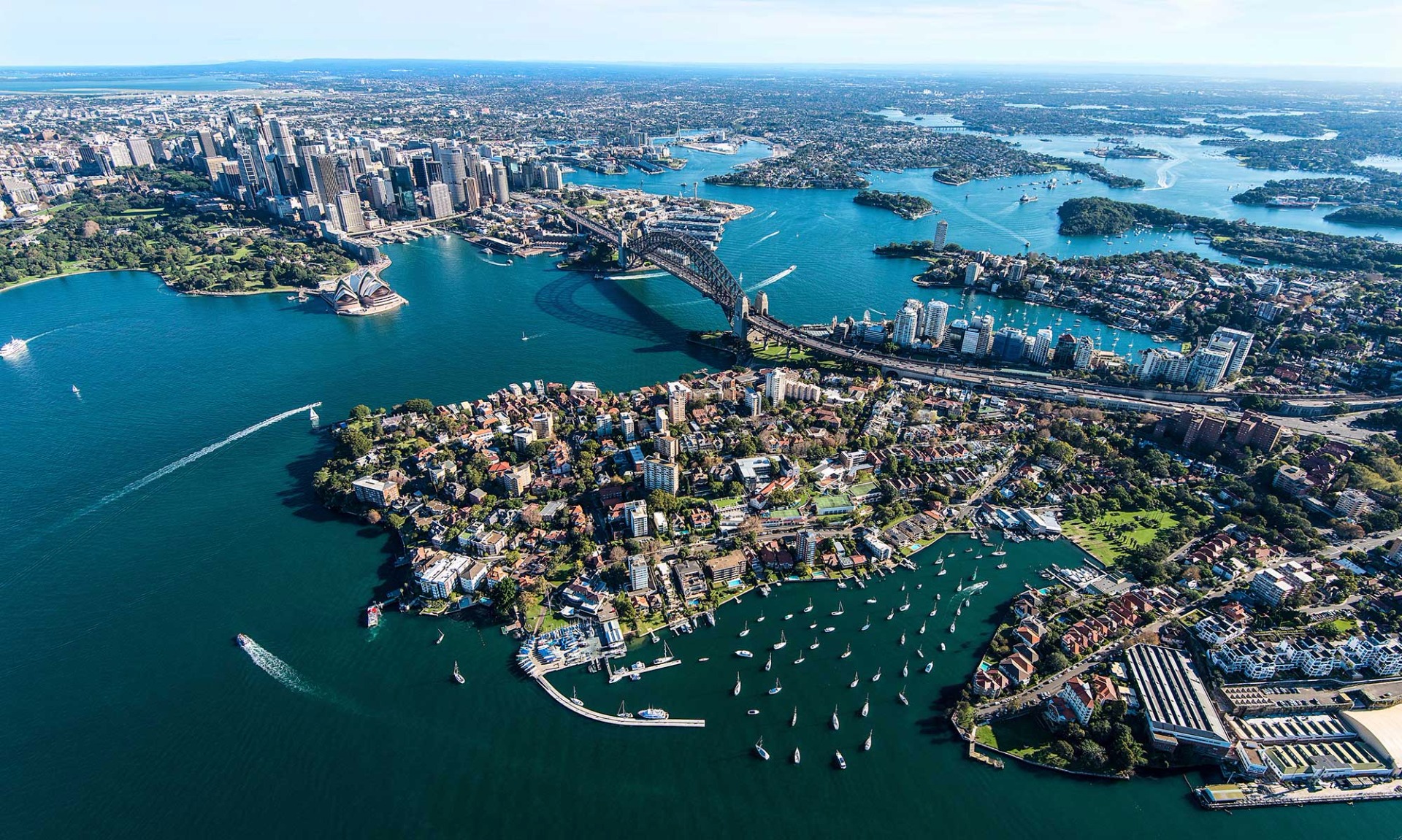This aerial photographic image captures a bustling metropolitan area characterized by multiple landmasses surrounded by blue and green waters. The city consists of interconnected islands and peninsulas, prominently linked by an arched bridge extending from the middle right towards the center of the image. Below, numerous boats traverse the water, leaving visible wakes of foam behind them. The foreground features a densely packed peninsula with a mix of white and brick buildings, giving way to taller skyscrapers and smaller homes further inland. In the distance, impressive gray skyscrapers define the horizon. The scene is animated with the vibrant activity of boats, diverse architectural structures, lush green areas, and a well-developed network of roads, including a significant highway leading to the bridge, uniting the varied elements of water and land.